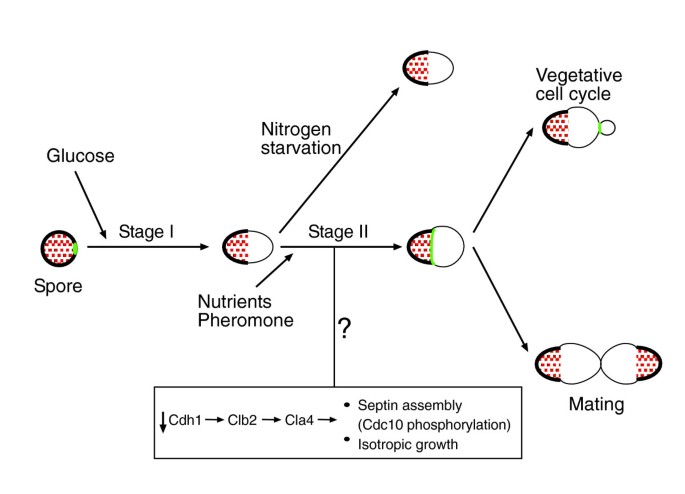The image depicts a detailed diagram on a white background illustrating the stages of spore development in response to various nutrients and conditions. At the upper left, a black circle with a red center labeled "spore" is present. An arrow pointing downward labeled "glucose" leads to "Stage 1", transitioning to an oval shape that is half white and half red, indicating the intake of nutrients and pheromones. This shape branches off to indicate different paths depending on nutrient availability - one arrow leads to "nitrogen starvation" and "Stage 2", continuing upwards to a black circle with a red center, surrounded by a green stripe and another white circle outlined in black. 

From here, there are two main pathways. The first pathway, leading upwards, is labeled "vegetative cell cycle" and is represented by another circular shape with red on the left side. The second pathway, leading downwards, follows a series of molecular interactions listed as CDH1 → CLB2 → CLA4, leading to septum assembly, CDC10 phosphorylation, and isotropic growth. This pathway is associated with another shape similar to an egg which then indicates the "mating" process.